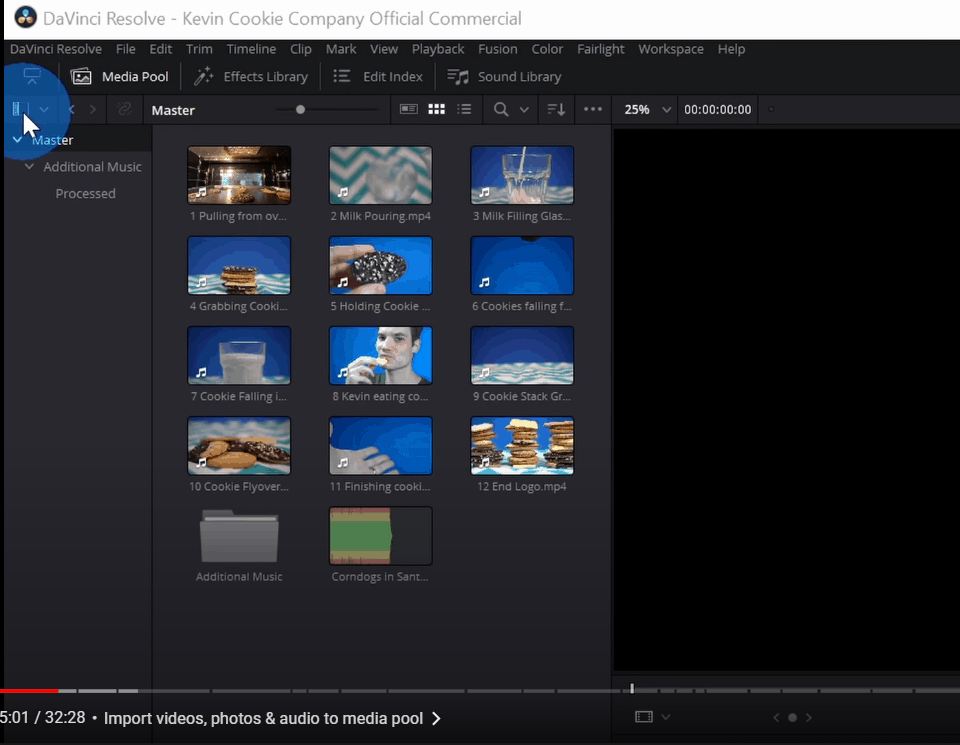In this detailed screenshot of the video editing software DaVinci Resolve, the interface is prominently shown as it appears during the editing of the "Kevin Cookie Company Official Commercial." At the top of the screen, a white title bar clearly states "DaVinci Resolve Kevin Cookie Company Official Commercial." Below this, the menu bar offers a comprehensive list of functions including File, Edit, Trim, Timeline, Clip, Mark, View, Playback, Fusion, Color, Fairlight, Workshop, and Help, all displayed in light gray against a darker gray background.

The software’s timeline at the bottom of the screenshot spans various chapters of the commercial, with each segment marked by timestamps and distinct labels. These segments are garnished with music icons and thumbnail shots, indicating different parts of the video content. A visible mouse cursor on the left side of the screen suggests interaction or movement within the video.

Further down, the status bar indicates "501 out of 3228," likely referencing frames or a specific point in the timeline, alongside import options for Videos, Photos, and Audio to the Media Pool. Slightly above the timeline, another utility bar includes options for Master, Search, and a zoom percentage set at 25%, along with the current timestamp. The layout is methodically organized, showcasing a clear and user-friendly workspace designed for efficient editing. This screenshot likely serves as a reference point, helping the user to remember a particular action during the video editing process.